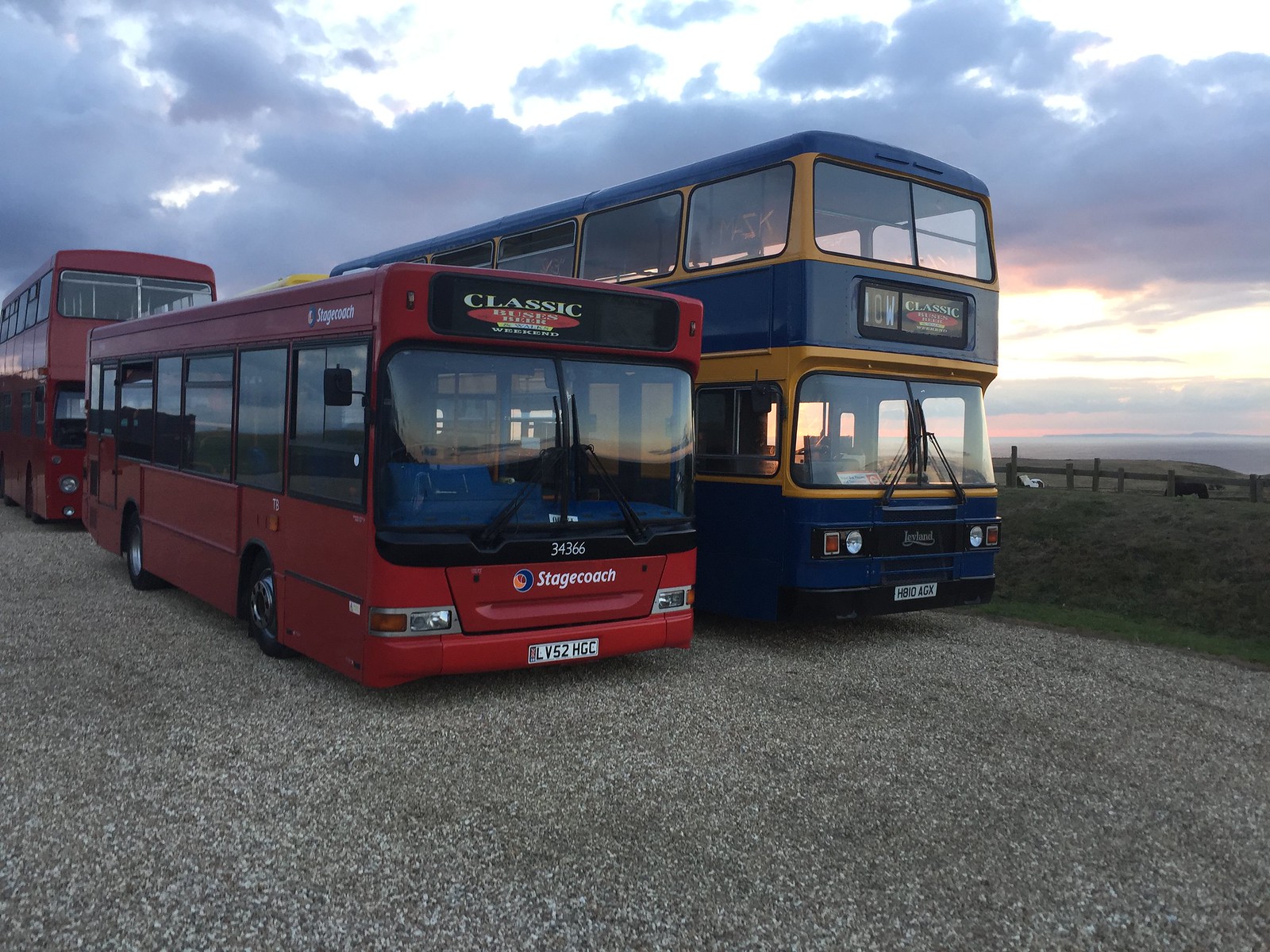A detailed photograph captures three buses parked outdoors on a gravel pathway. At the forefront is a bright red single-decker bus, prominently displaying the word 'Stagecoach' in white italicized letters. Above its large windows, a sign reads 'Classic.' Adjacent to it is a striking double-decker bus donning a navy blue and yellow color scheme, with distinctive signage on its front. Behind these two, another red double-decker bus with expansive windows completes the trio. The gravel pathway they rest upon is bordered by a green field, where a fence lines the boundary, and two animals, likely cows or horses, graze peacefully in the distance. The landscape gently rises to the right, marked by wooden posts. Overhead, a sky dense with puffy gray clouds is pierced by the sun, casting a bright but subdued light, suggesting either dawn or dusk. The scene is devoid of people, adding to the sense of stillness and tranquility. The license plates of the buses, LV52HGC on the front red bus and H210AGK on the blue and yellow double-decker, add a touch of specificity to this serene snapshot.